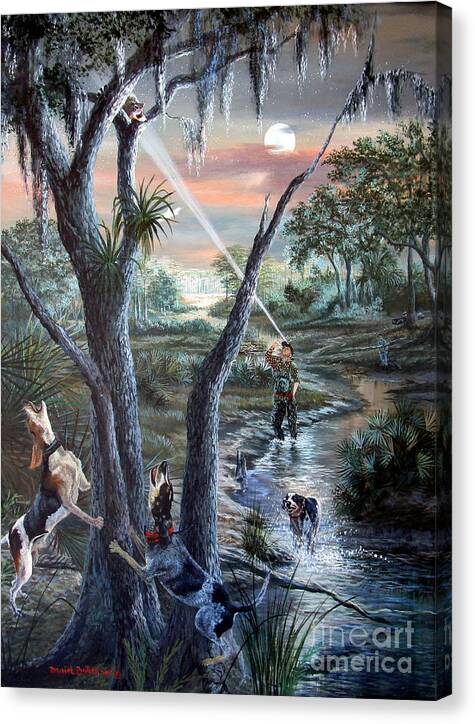In this modern semi-realistic painting, we observe a nocturnal hunt set within a dense, forested swamp under a night sky. A partially obscured full moon, emitting a white glow, peeks through a canopy of red, blue, and grey clouds. A man, donning a cap with an affixed flashlight, stands knee-deep in the river. His beam of light illuminates an indistinguishable animal perched high in a tree. At the base of this tree, situated towards the left side of the canvas, three dogs energetically bark upwards — two are at the foot of the tree, while one stands in the river behind them. The surrounding scene is lush with vegetation, including ferns and various other flora. The background features several other trees, enhancing the dense and forested ambiance. In the bottom right corner of the image, the text "Fine Art America" is clearly inscribed in white.